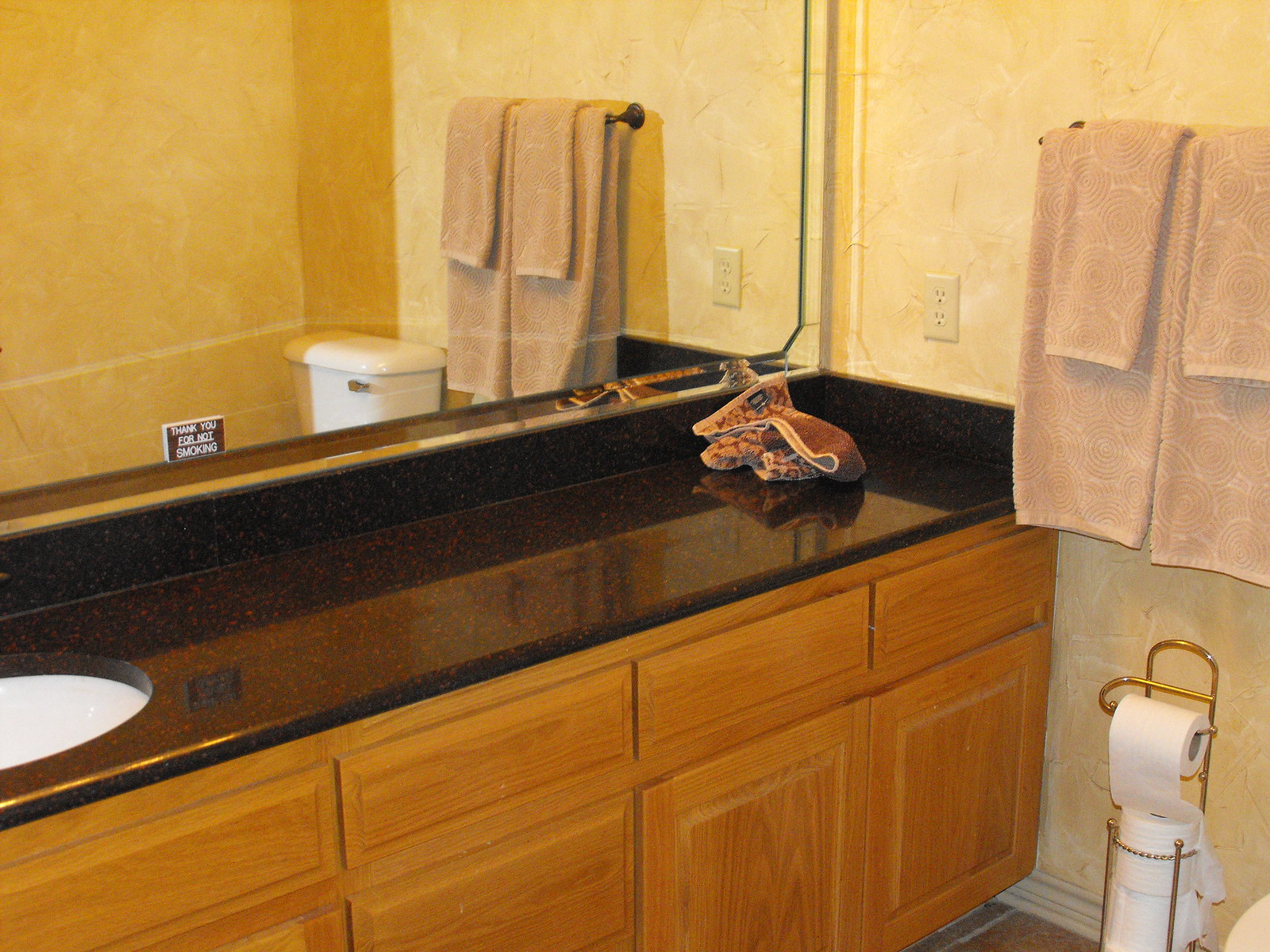A detailed depiction of a bathroom in a possible restaurant setting. The scene prominently features a counter and sink area with a thoughtful layout and design elements. On the upper left side of the image, occupying about a third of the picture, is a mirror. Reflected in this mirror are two towels, an electrical socket without safety covers, a toilet, and a small plaque with the message "Thank you for not smoking," suggesting this could be a restroom in a restaurant.

The sink is crafted from black and red marble and is positioned to the far left. The counter itself lacks drawers but consists of three separate segments designed for storage. To the left of the counter is a wall with a marble design, although it appears to be made of polyester. 

On the right side of the counter are additional towels, also visible in the mirror, along with a brass holder that dispenses a single horizontal toilet paper roll and provides space below for storing two extra rolls. The floor is adorned with tiles in a brown and burgundy color scheme, adding to the rich aesthetic of the room.